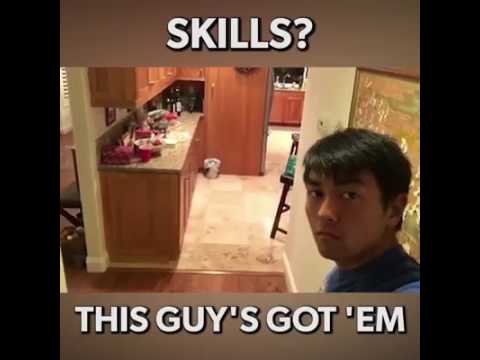In the image, a young man stands in a central, indoor setting, likely a kitchen. He is positioned slightly to the bottom right and looks directly at the camera with a confident or questioning expression. The background reveals a kitchen with wooden cabinets, countertops cluttered with various items, a combination of hardwood and tile flooring, and multiple colors including brown, tan, black, white, green, red, and yellow. The man, who appears to be of Asian, Native American, or Hispanic descent, has black hair and brown skin. The image is bordered in solid black and features the text "Skills. This guy's got them" at the top, suggesting it’s styled as a shareable meme. The overall image hints at showcasing the man's skills, though the specific nature of these skills is unclear.